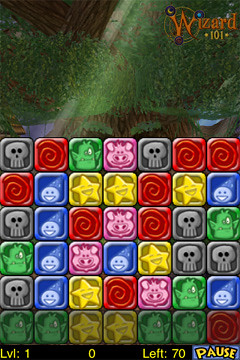This image showcases gameplay from a video game. On the top right corner, "Wizard" is prominently displayed in orange text, with "101" written just below in yellow. In the bottom left corner, the text "LVI:1" appears, followed by a zero in the middle. On the bottom right, "Left: 70" is visible in yellow text, alongside the word "Pause".

The central focus of the image features an array of square blocks, each adorned with unique designs and colors. Among these blocks, several stand out: one block displays a red spiral design, another in dull gray represents a school theme, and a yellow block is marked with a star design. The variability in the block patterns highlights the game's intricate and visually engaging environment.